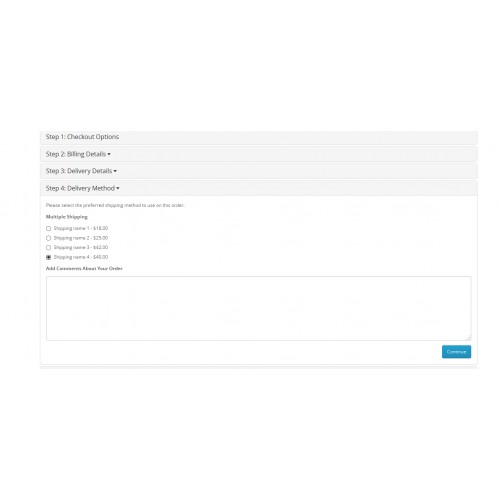The image depicts a small rectangular box with a light gray outline. At the top of the rectangle, there are four horizontal lines in a slightly darker gray shade, each containing text that is too small to read. These lines are labeled on the right-hand side as Step One, Step Two, Step Three, and Step Four, although the accompanying descriptive text beside these labels is unreadable.

Below these initial lines are three more rows, each accompanied by small dots next to the labels Step Two, Step Three, and Step Four. Again, the text next to these steps is too small to decipher. Underneath these rows is another section of text in very small white print, enclosed within a light gray outline filled with white. This section also contains unreadable words.

Further down, there are four circles, three of which are outlined in gray, while the bottom circle is filled in black. Each circle has text beside it, but the text is too small to see clearly. At the very bottom of the rectangle is a smaller gray-outlined box that appears intended for information input.

Finally, in the lower right-hand corner of the whole setup, there is a blue box with white writing that is also too small to read.